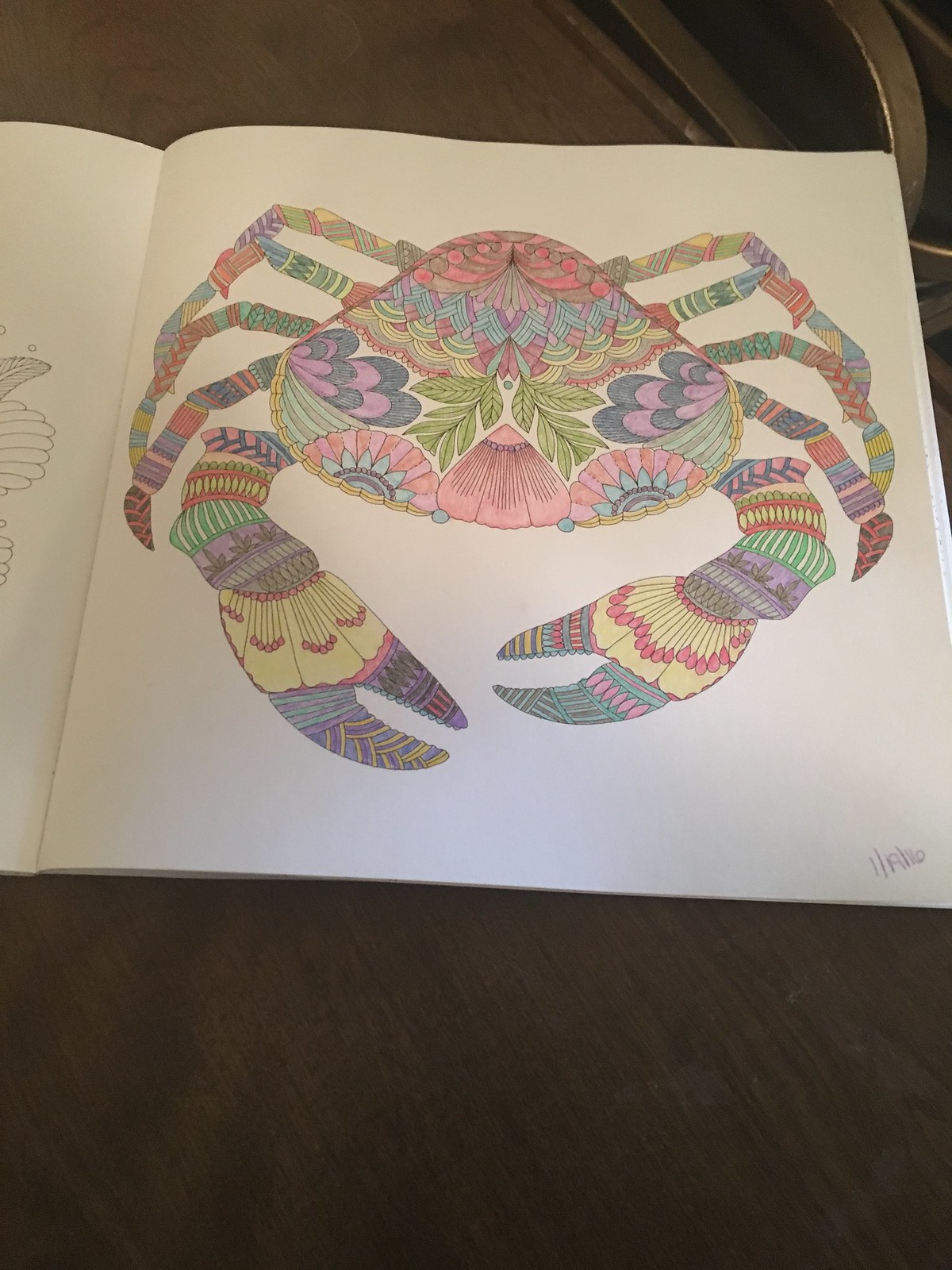In this vibrant and detailed sketch, a colorful crab takes center stage, presented on what appears to be a page from a coloring book or notebook. The crab is depicted from a frontal viewpoint, showcasing its intricate and vividly colored features. Positioned at the bottom of the image is a dark gray sheet, reminiscent of a bed or couch cover, providing a stark contrast to the dynamic hues above.

The crab exhibits a full spectrum of colors, with its claws, legs, and body adorned in various patterns of lines. The eight legs, extending in the background, and the vividly ornate claws are particularly eye-catching, reflecting every shade of the rainbow. To the left edge of the page, another sheet peeks out, displaying just the outer sketch of the crab's design, hinting at the process of coloring and the artistic creativity involved in bringing this aquatic creature to life.